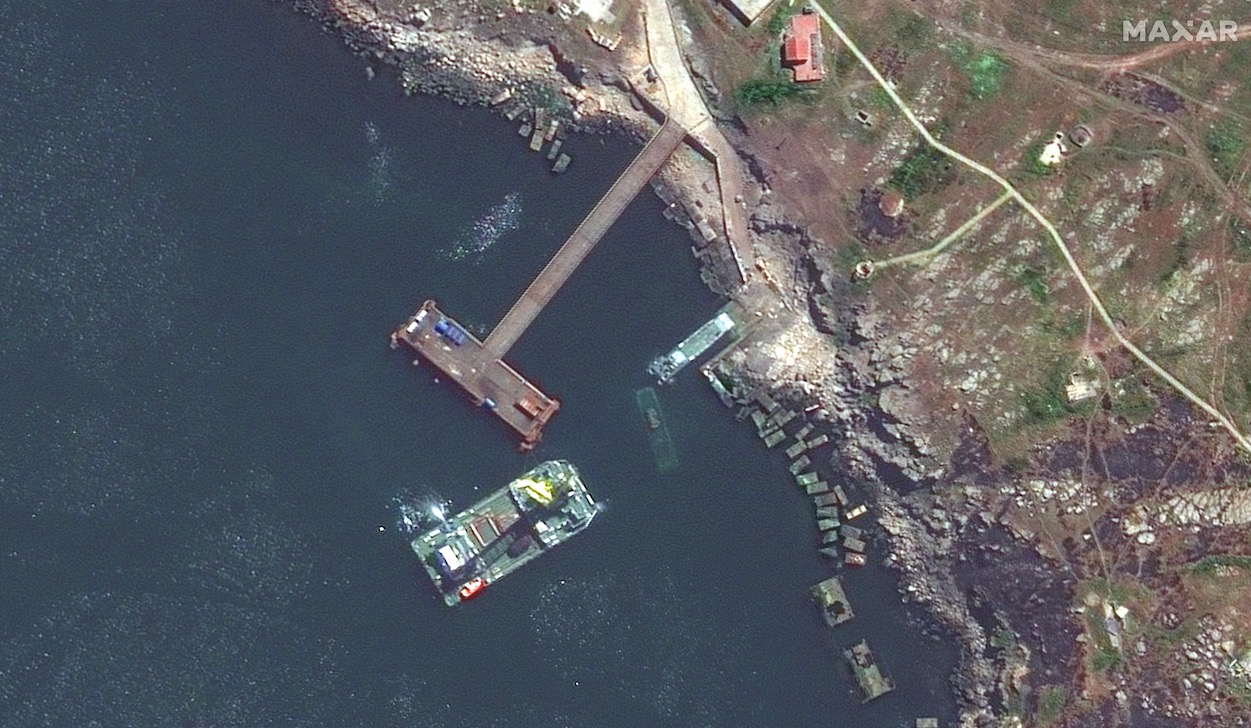This aerial photograph captures a stark, arid landscape featuring a coastal area with a prominent dock extending into dull grayish-blue water. Numerous boats or barges, including a long rectangular one with what appears to be a connecting bridge, are scattered across the water, surrounded by small, box-like objects that could be cargo or debris. The shoreline is rocky and predominantly brown, with dry, leafless terrain mixing sporadically with patches of green. The landscape includes various roads, including a whitish main road and a wider access road leading directly to the dock. Overlooking the craggy shoreline, a notable red-roofed building stands out, with another smaller building with a red roof visible at the top edge of the image. The upper right corner of the photo is marked with the watermark "Maxar."